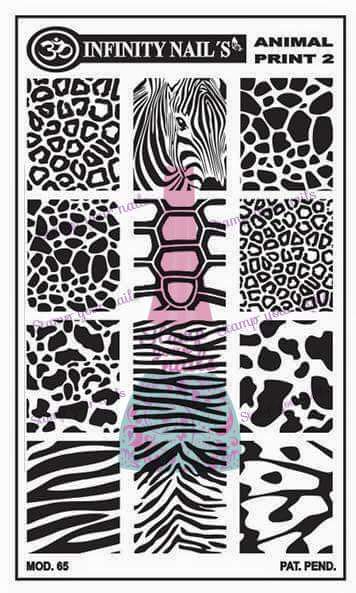The image is a detailed poster primarily in black and white with some splashes of color. At the top, it features "Infinity Nails" written in white text on a black rectangular background. To the right, "Animal Print 2" is displayed in black text. The central part of the poster showcases 12 different rectangular designs with various animal prints, mostly in black and white, including patterns resembling zebra and cheetah skins. Some designs incorporate colors, with one featuring pink and another blue. Additional details include "MOD.65" written in the bottom left corner and "PAT.PEND" in the bottom right corner. The poster appears intended to showcase nail decal designs.